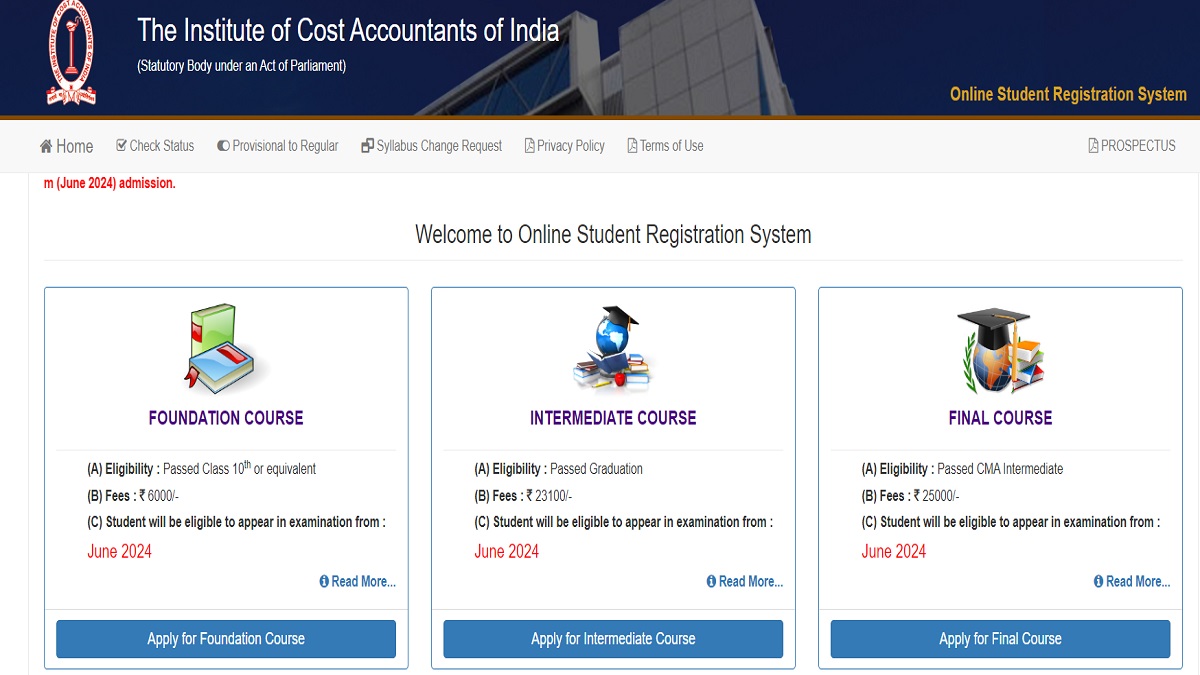This is an image showcasing the homepage of the Institute of Cost Accountants of India's website. The top section features a dark blue bar with the institute's name in white font, "Institute of Cost Accountants of India", followed by a smaller parenthetical text "Statutory body under an Act of Parliament". On the left side of this bar is the institute's logo - a white seal shape adorned with a banner and a star at the bottom. On the right side of the bar, in gold font, it reads "Online Student Registration System".

The main body of the webpage has a white background. Directly below the dark blue bar is a navigation menu featuring links such as "Home", "Check Status", "Provisional to Regular", "Syllabus Change Request", "Privacy Policy", and "Terms of Use". On the right, there is an additional link labeled "Prospectus". Beneath this, in red font, it states "M", followed by "June 2024" in parentheses, and a small font notation "mission".

Centrally displayed in black font is a welcoming message: "Welcome to Online Student Registration System". Below this, the page is divided into three blocks, each representing different courses offered by the institute. 

1. **Foundation Course**:
   - Accompanied by a cute icon with two books (a green upright book and a blue book lying down).
   - Eligibility: Passed class 10th or equivalent.
   - Fees: 6,000 (currency unspecified).
   - Students will be eligible to appear in the examination from June 2024 (this date is highlighted in red).
   - There is a "Read More" link and a blue "Apply for Foundation Course" button in white font.

2. **Intermediate Course**:
   - Eligibility: Passed graduation.
   - Fees: 23,100 (currency unspecified).
   - Students will be eligible to appear in the examination from June 2024.
   - Contains a "Read More" link and a blue "Apply for Intermediate Course" button in white font.

3. **Final Course**:
   - Eligibility: Passed CMA Intermediate.
   - Fees: 25,000 (currency unspecified).
   - Students will be eligible to appear in the examination from June 2024.
   - Includes a "Read More" link and a blue "Apply for Final Course" button in white font.

Each course block provides essential eligibility criteria, fees, and examination eligibility timeline, along with options to read more details or apply directly.